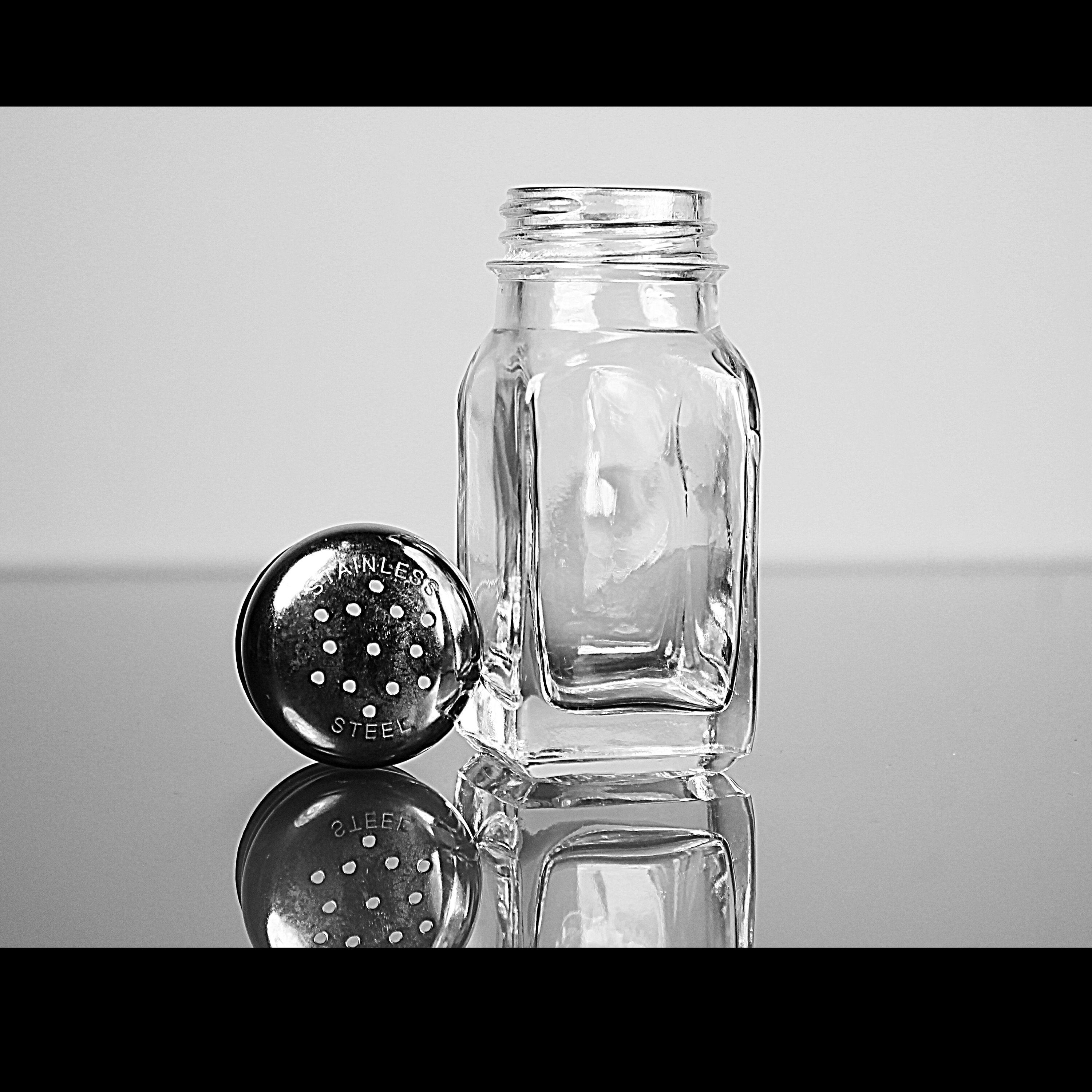This image features a premium glass salt shaker, positioned prominently on a glossy silver-like surface that reflects the shaker beneath. The photograph is characterized by letterbox-style black bars at both the top and bottom, suggesting it could be a screenshot from a video. The background is an indistinct whitish-gray, possibly appearing light blue or white depending on the lighting. The clear, thick glass bottle of the salt shaker is square at the bottom and rounded at the top, with the cap, which is placed separately to the left, made of shiny stainless steel and labeled as such. The cap, featuring small holes for dispensing salt, illustrates a quality finish, hinting at the image's promotional intent. The entire composition is captured at eye level, creating a professional and presentable display of the product.